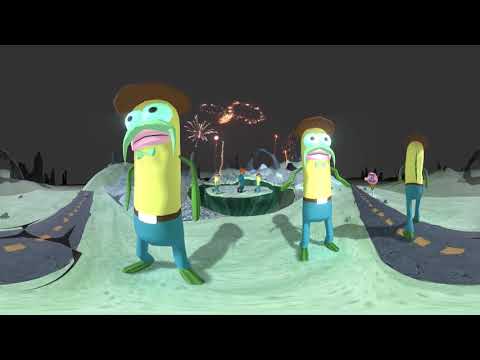The image displays a vibrant, early-2000s style 3D rendering of a colorful, whimsical game world. The scene features two intersecting roads, each with a dotted yellow line running down the center, and light gray-to-green terrain on either side. In the foreground stands a pair of identical, oblong fish-like characters. These characters have green fins for feet and limbs, white mustaches, googly eyes, and brown cowboy hats. They are adorned with brown belts, enhancing their quirky appearance. Additional identical characters populate the scene, creating a playful, uniform vibe. One unique character sports a green shirt and red hair. Further back, a pink character is visible near a circle, flanked by aquatic-looking plants and green terrain. In the distance, multiple hills rise against a dark gray skybox, punctuated by three red fireworks exploding, adding a festive touch to the surreal landscape.